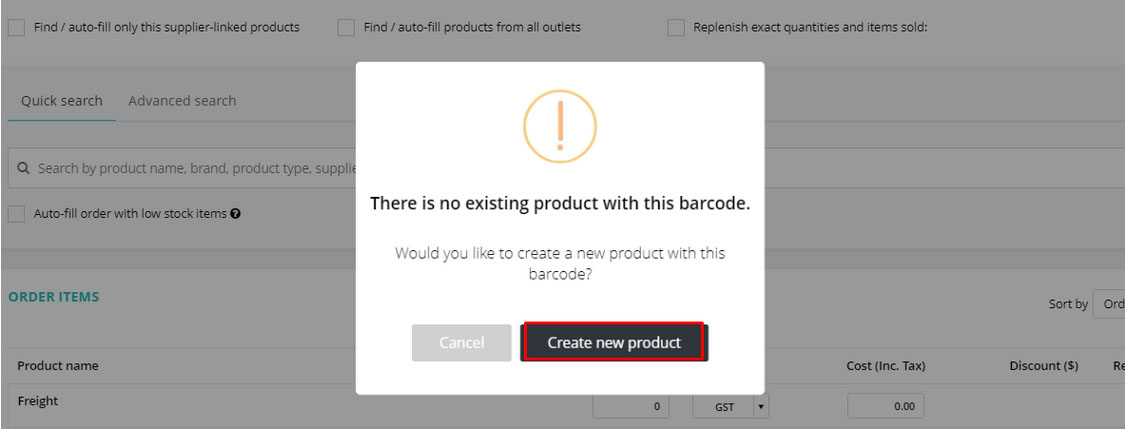The image depicts a barcode search interface. In the top left corner, there are three unchecked boxes with the following labels: "find autofill only this supplier linked products," "find autofill products from all outlets," and "replenish exact quantities in items sold." Below these options, there is an underlined "Quick Search" link followed by an "Advanced Search" link. 

Further down, there is a search bar featuring a magnifying glass icon and the prompt, "Search by product name, brand, product type, supply," which is partially obscured by an overlaid image. Nearby, another unchecked box is labeled "autofill order with low stock items," followed by a question mark icon. 

The section underneath is titled "Order Items," followed by "Product Name" and "Freight." In the middle of the page, part of the content is obscured by a white square overlay. At the top of this square, there is a circular icon with an orange border, containing a large exclamation point. The message within the white square reads: "There is no existing product with this barcode. Would you like to create a new product with this barcode?" Below this message, there are two buttons: a gray rectangle labeled "Cancel" and a black rectangle with a red border labeled "Create New Product."